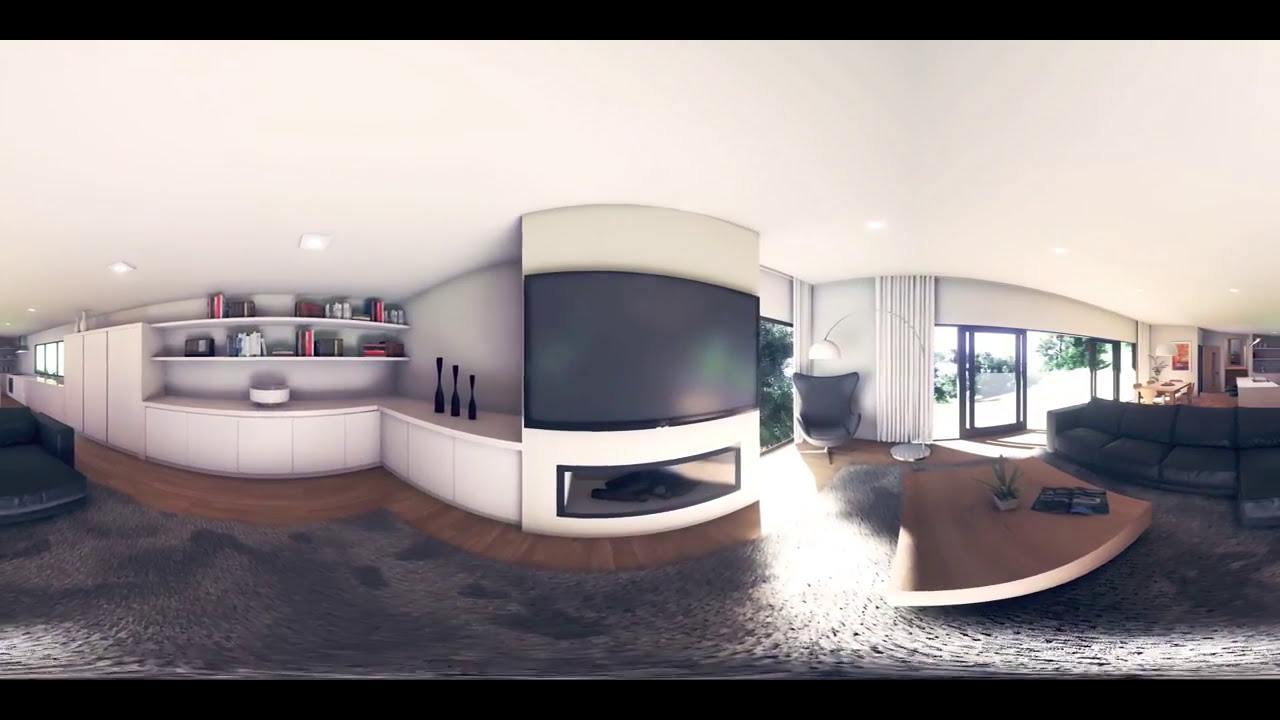The image depicts a modernistic living area captured in a 360-degree panoramic view. Central to the room is a large, wall-mounted flatscreen TV on a white stand. The left side features white countertops, shelves, and cabinets, filled with decorative items, books, and kitchen appliances like a toaster and coffee machine. The shiny, black tiled floor transitions into a rich hardwood plank floor as you move towards the right side of the room. Right of the TV, a luxurious black leather sectional sofa sprawls, complemented by a modern black recliner with a white lamp overhead. A contemporary brown coffee table adorned with a plant and magazines sits in front of the sofa. Extended sliding glass doors and wall-to-wall windows on one side illuminate the room. The overall aesthetic is distinctly modern with a blend of hardwood, carpet, and advanced electronic features, making the space appear both stylish and functional.